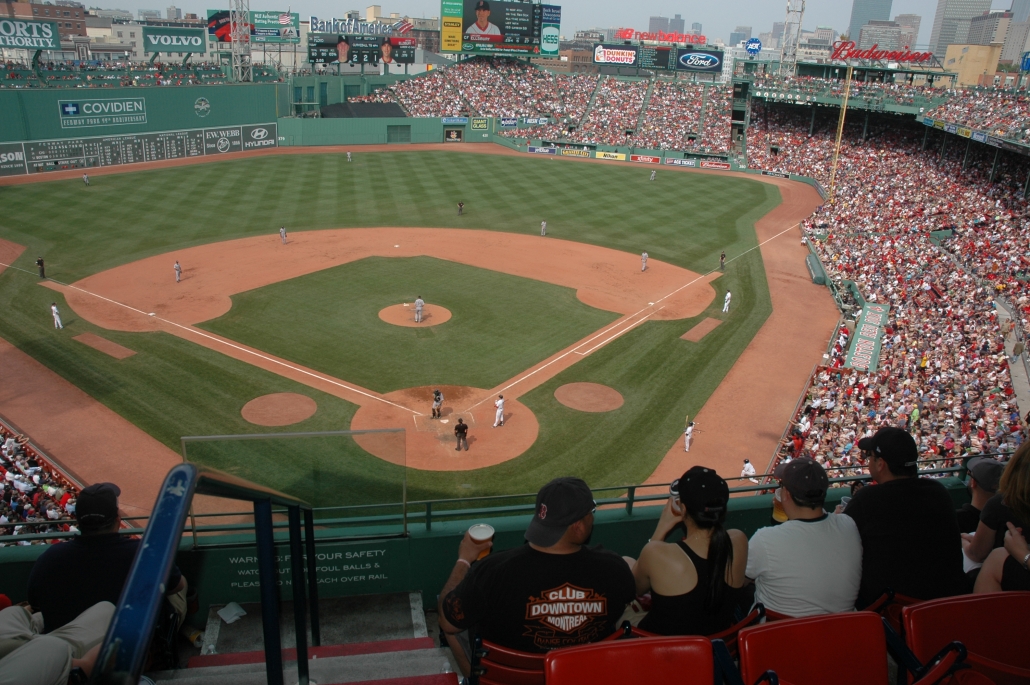The photograph captures a vibrant baseball game from a vantage point high up in the bleachers, close to the nosebleed seats, behind home plate. In the foreground, four spectators are seated in red chairs: a man with a backward baseball cap, a girl with a ponytail wearing a black hat and black top, a man in a white shirt and a baseball cap, and another man in a dark shirt and black cap. The stadium is packed with fans, a sea of reds and whites. All the players are on the field, dressed in white, with a pitcher at the center, a catcher, and an umpire visible. No one occupies the bases, but a batter is stepping up to the plate. The scene is bustling with corporate advertisements, including notable brands like Budweiser, Bank of America, Volvo, Dunkin Donuts, Ford, and Sports Authority. The clear sky above and tall skyscrapers in the background add to the atmosphere of an exciting, well-attended game.